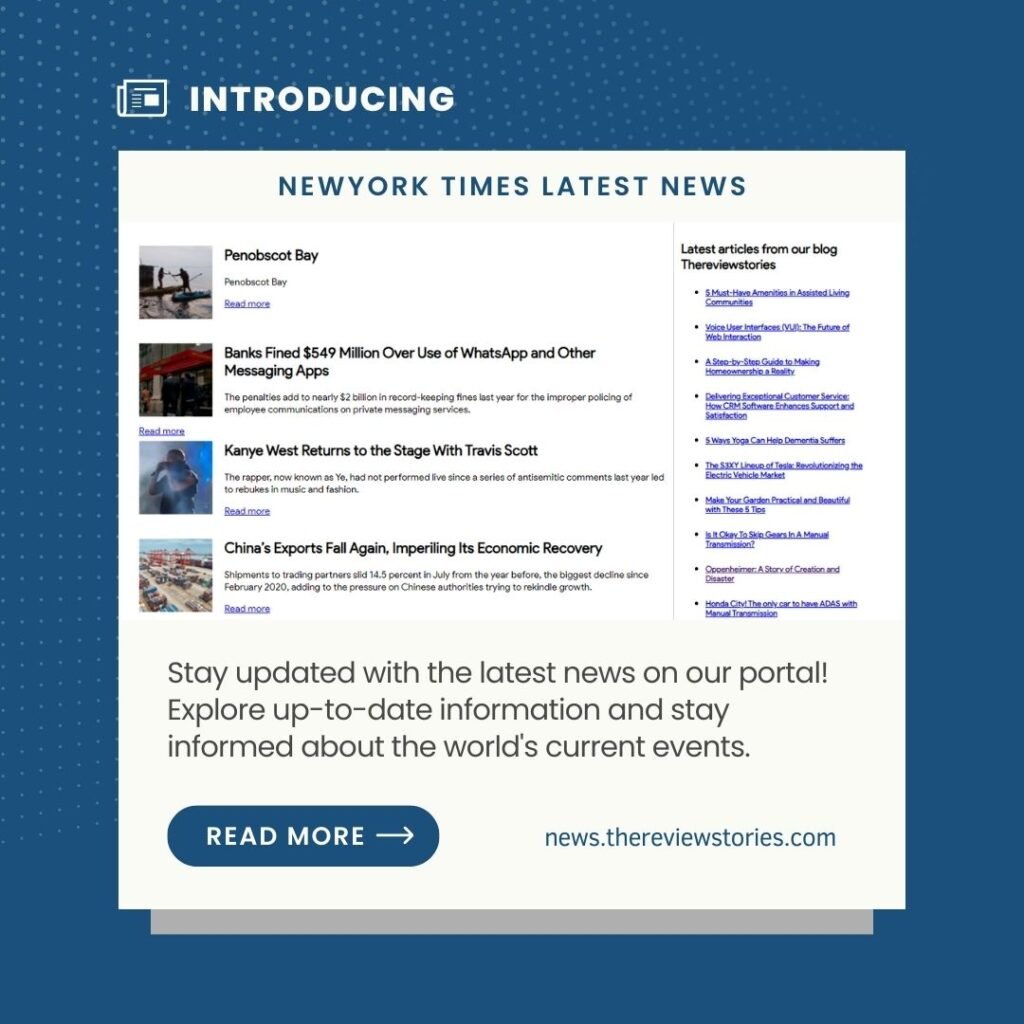**Introducing the Latest from Texas A&M University: Stay Informed with New York Times, Penobscot Bay News, and More**

On a blue background, the highlights include:

- **Texas A&M University**
- **New York Times Latest News**
- **Penobscot Bay** featured prominently twice.
- **Interactive Elements**: Options to "Read More" and "Just Read Something".

Key Content Areas:

1. **Latest Articles from Our Blog**:
    - **Reviews and Voice User Interfaces**: Detailed insights and step-by-step guides on developing exceptional customer services.
    - **Social Media, Software Support and Satisfaction**: Exploring trends and best practices.
    - **Wellness**: Yoga as a potential aid for sufferers of various conditions.

2. **Major News Stories**:
    - **Bing Fined $549 Million**: Over WhatsApp and other messaging app usage. Total penalties approach nearly $2 billion due to record-keeping, privacy, and public communication issues.
    - **Kanye West Returns**: The artist, now known as "Ye," sets the stage after a hiatus following anticipated call-outs last year.
    - **China's Economic Update**: Exports decline with a 25% drop in July year-over-year, marking the biggest fall since February 2020. Increased international pressure aims for China’s growth.

Also featuring continuous updates to stay informed with the latest news and events worldwide. Look for additional tags and resources such as "Texas A&M News", "Tarleton Reviews", and "Tories.com", all set against a neutral grey background for easy navigation and reading.

---

Stay connected and updated with the most recent and relevant information provided for an enriched understanding of current affairs.